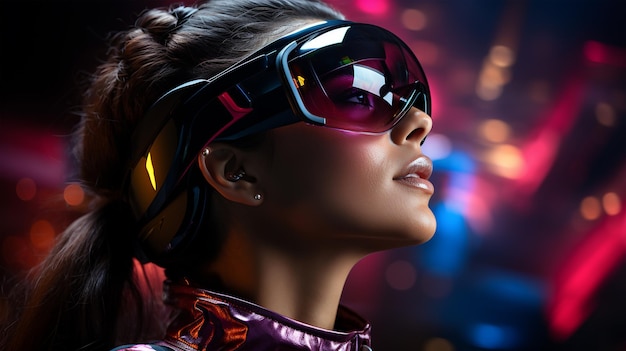The photograph captures a striking headshot of a black woman, exuding a futuristic and warrior-like aura. She is modeling large, semi-transparent VR goggles with a maroon, almost pinkish-reddish tint. The goggles, which resemble ski goggles in size, feature a thick, black strap with hints of yellow that securely wraps around the back of her head, where her brown hair is styled in a braid.

Her face is partly visible through the tinted, rose-colored lenses, and she is adorned with subtle makeup, including pink lipstick, enhancing her confident expression. Tiny earrings and two tattoos—one on her earlobe and another on the conch of her ear—add unique details to her appearance.

She is dressed in a shiny, metallic, silver-gray turtleneck jacket that zips up high around her neck, reminiscent of an astronaut's suit. The highly reflective material of her outfit adds to the avant-garde feel of the image.

The background is a blur of vibrant colors—orange, red, blue, and black—sparkling and suggesting stage lights or a digitally enhanced environment, enhancing the impression that she might be part of a VR game or futuristic scene. The lights create dynamic reflections on her goggles, further enriching the highly polished and professional look of the photograph.